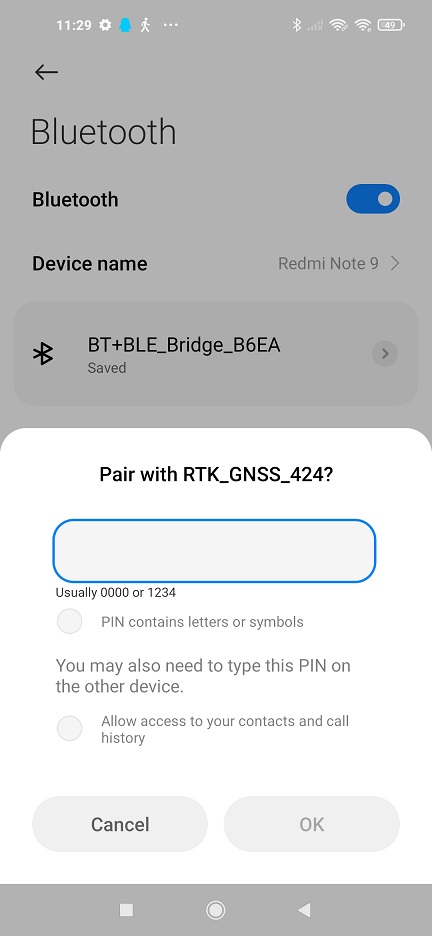A screenshot from a Redmi Note 9 smartphone displays a Bluetooth pairing screen. The time shown on the phone is 11:29, and the battery level is at 49%, with a strong signal strength indicated. The background of the screen is predominantly gray. 

At the top-left corner, a black arrow points to the left, accompanied by the text "Bluetooth" displayed twice, signifying that Bluetooth is turned on. The device name "Redmi Note 9" is visible, with detailed information provided underneath: "BT + BLE_BRIDGE_B6EA," followed by the status "saved."

The pairing section is set against a white background and suggests pairing with "RTK_GNSS_424?" There is a blue text box present, typically used for entering a PIN, with the note "usually 0000 or 1234" beneath it. It also contains a gray instruction circle stating, "PIN contains letters or symbols," highlighting that additional complexity in the PIN may be required.

Further down, there's information suggesting that the user might need to enter this PIN on the other device as well, alongside an option to "allow access to your contacts and call history." At the bottom of the screen, there are two action buttons: a gray "Cancel" button with black text and an "OK" button, indicating that the user canceled the pairing process. Below these elements, the standard Android navigation buttons for "Close," "Home," and "Back" are visible.